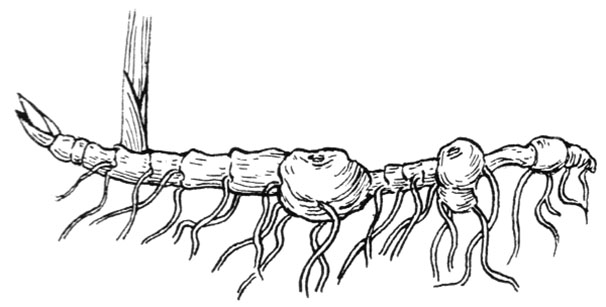This black-and-white illustration, possibly a pen and ink drawing, appears to depict an ambiguous hybrid form that could belong to either the botanical or zoological world. The main structure is long, segmented, and horizontally oriented, resembling either a twig or an elongated insect. Each segment has varied textures and ridges, enhancing the detail of its narrow-to-wider contour transitions. Dangling from the bottom of the segments are appendages that evoke the image of either roots or jellyfish-like tentacles, amplifying the uncertainty about its true nature. 

The far end of the structure features V-shaped elements that could be interpreted as budding leaves. At the very end, a projection rises upwards, similar to a small column or poles. Despite the enigmatic head or tail-like formation at the front, identifying its face or definitive beginning is challenging due to the side view angle. This image, with its intricate detailing and the stark contrast against a blank background, could easily belong in a science textbook, inviting viewers to ponder its identity and classification.